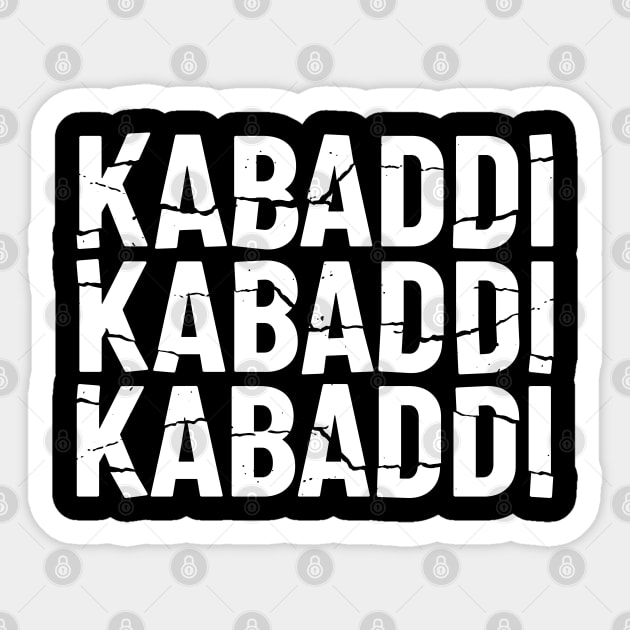The image features a digital sticker design over a gray background adorned with a pattern consisting of gray circles, each containing a white twisted padlock symbol. These circles are connected by diagonal lines, creating a diamond-shaped lattice throughout the backdrop. In the center of the image, a prominent white-bordered sticker stands out. This center sticker has a slightly wavy outline and encloses a black background. Written across this black section in large, bold, capital white letters is the word "Kabaddi" repeated three times, each word aligned in a column. The text appears as if it is cracked or crumbling, adding a distressed effect. The overall design gives a modern and edgy feel, combining geometric patterns with a distinctive central motif.